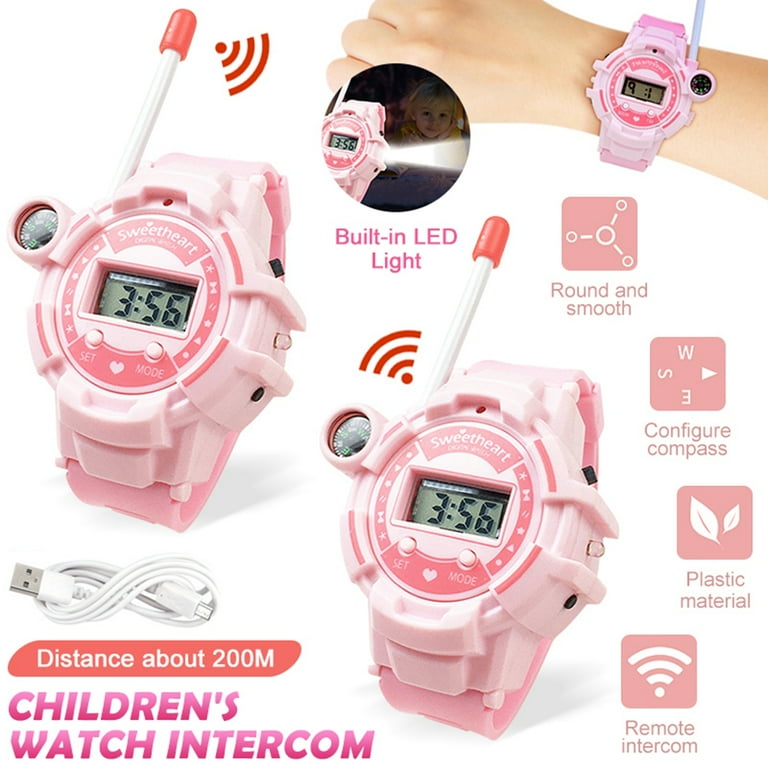The advertisement features a high-tech children's sports watch, predominantly pink with accents of darker pink and a digital LCD display. The watch, large and robust in design, includes an extendable antenna with a red tip and a built-in compass. The image highlights multiple perspectives: a close-up of the watch on a small child's wrist at the top right, and additional close-ups in the center and bottom sections of the ad. Text at the bottom left states "Distance about 200 meters" and "Children's Watch Intercom." Icons surrounding the watch detail its features—highlighting its round and smooth design, built-in LED light, plastic material, and remote intercom capabilities. The word "Sweetheart" is displayed prominently at the top of the watch face. A small circled inset shows a girl demonstrating the LED light feature. The right side of the advertisement lists the watch's key attributes: round and smooth, configure compass, plastic material, and remote intercom.